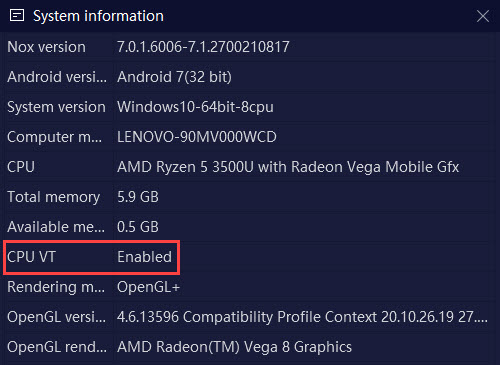The screenshot depicts a cropped selection from a specific tab on a computer, revealing the system information profile. Within this window, various details about the current system are displayed. The Nox version lists a serial number, while the Android version is identified as Android 7 32-bit. The system is running Windows 10 64-bit AECPU, and the computer model is a Lenovo equipped with an AMD Ryzen 5 3500U CPU. The total memory available is 5.9 GB, with 0.5 GB currently available. Notably, the section for CPU VT is highlighted with a red box and is shown as enabled. Additionally, there are three categories related to rendering: OpenGL version and OpenGL rendering.